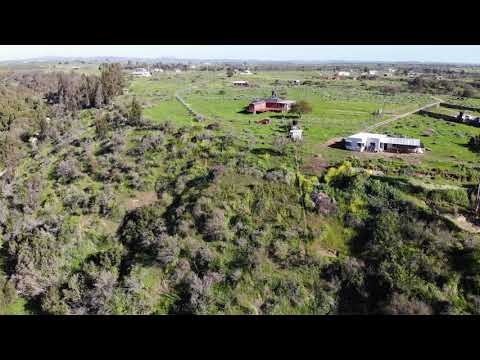An aerial view of a rural neighborhood captured from above, framed by thick black lines at the top and bottom of the image. The landscape predominantly features a lush expanse of green foliage, including a variety of trees, bushes, and grasses interspersed with red and yellow hues. In the upper middle of the photo stands a salmon-colored house with a gray roof, situated amidst a green field. To its right, there's a long, mostly white building that resembles either a large trailer or motorhome at the end of a dirt road. Further back on the right, another small, white house is visible against the backdrop of green fields and dense trees. The horizon is marked by a strip of white sky, possibly with faint mountain or town scenery in the distance. The serene, expansive landscape underscores the rural and predominantly undeveloped character of the area.